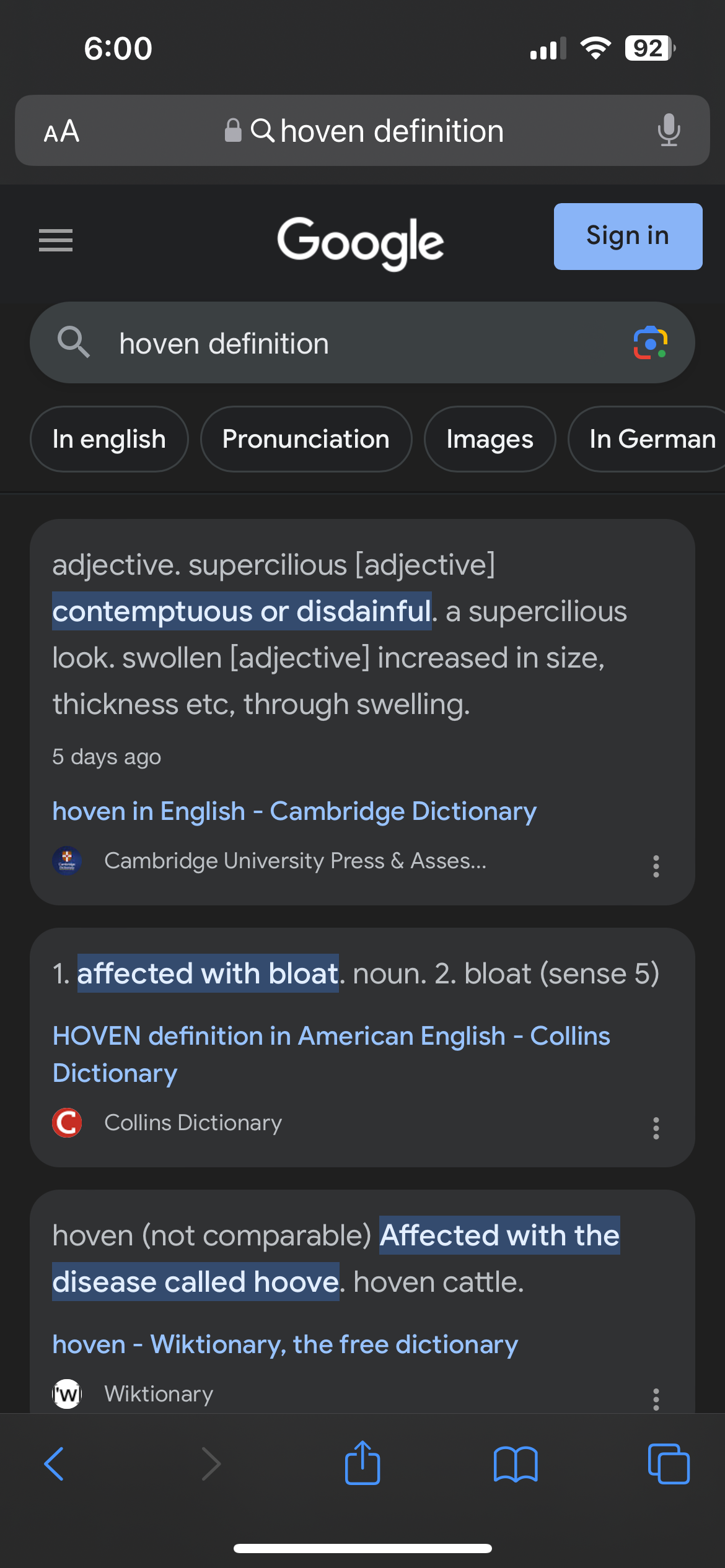The image displayed on the phone shows a Google search results page with the query "Hoven Definition." The phone's battery is at 92%, connection strength is indicated by 3 out of 4 bars, and the time is 6:00. At the top of the screen, the Google logo appears in white with a blue "Sign in" button to the right. Below the search bar, which again displays "Hoven Definition," there is a phonetic guide for English pronunciation, and options to view images in German.

The search results include multiple entries:

1. A definition from an unspecified source, describing "hoven" as an adjective meaning supercilious, contemptuous, or disdainful, and also as swollen, defined as increased in size or thickness through swelling.
   
2. A post made 5 days ago again mentions "hoven" and directs to the English definition in the Cambridge Dictionary, explained as "affected with bloat" with the noun form being "bloat."

3. An entry from the Collins Dictionary with "Sense 5" related to "Hoven Definition in American English."

4. A description indicating "hoven" is not comparable, affected by a disease called Hovi, with a reference to "hoven cattle" on Wiktionary, the free dictionary.

At the bottom of the screen, standard navigation icons for the phone interface are visible.